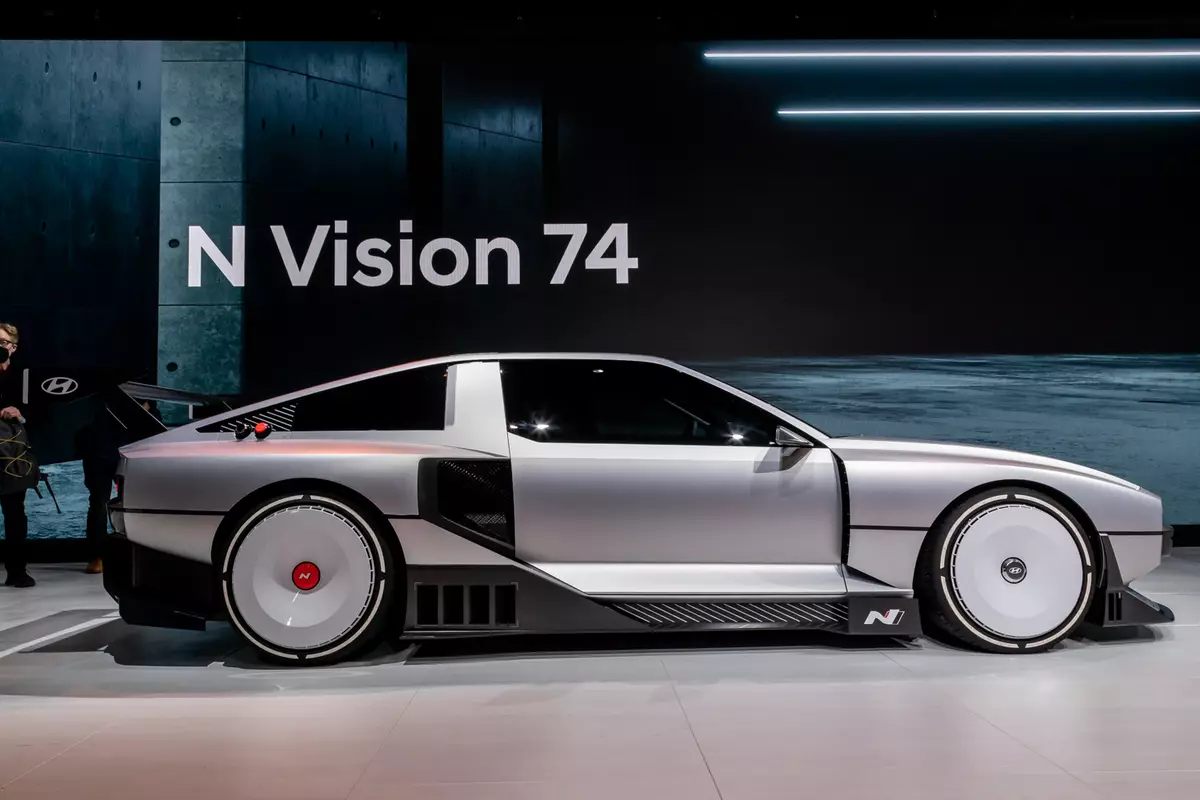The image showcases a futuristic prototype car in a sleek showroom or garage. The car is predominantly silver with solid silver hubcaps and low-profile black tires adorned with four distinct white borders that do not touch. Emblazoned on the top of the car is "N Vision 74," along with another prominent 'N' on its side. The vehicle, which resembles a sporty, low-to-the-ground two-door design, possibly akin to a Porsche, features extremely tinted windows and a rear spoiler. A Hyundai logo is visible, indicating the brand. Additionally, the back rear tire's center cap is notably red, while the front tire cap remains silver. To the side of the car, a man wearing a black mask is seen holding an unidentified object. The car's appearance and the showroom's advanced lighting suggest a modern, perhaps even futuristic, aesthetic.